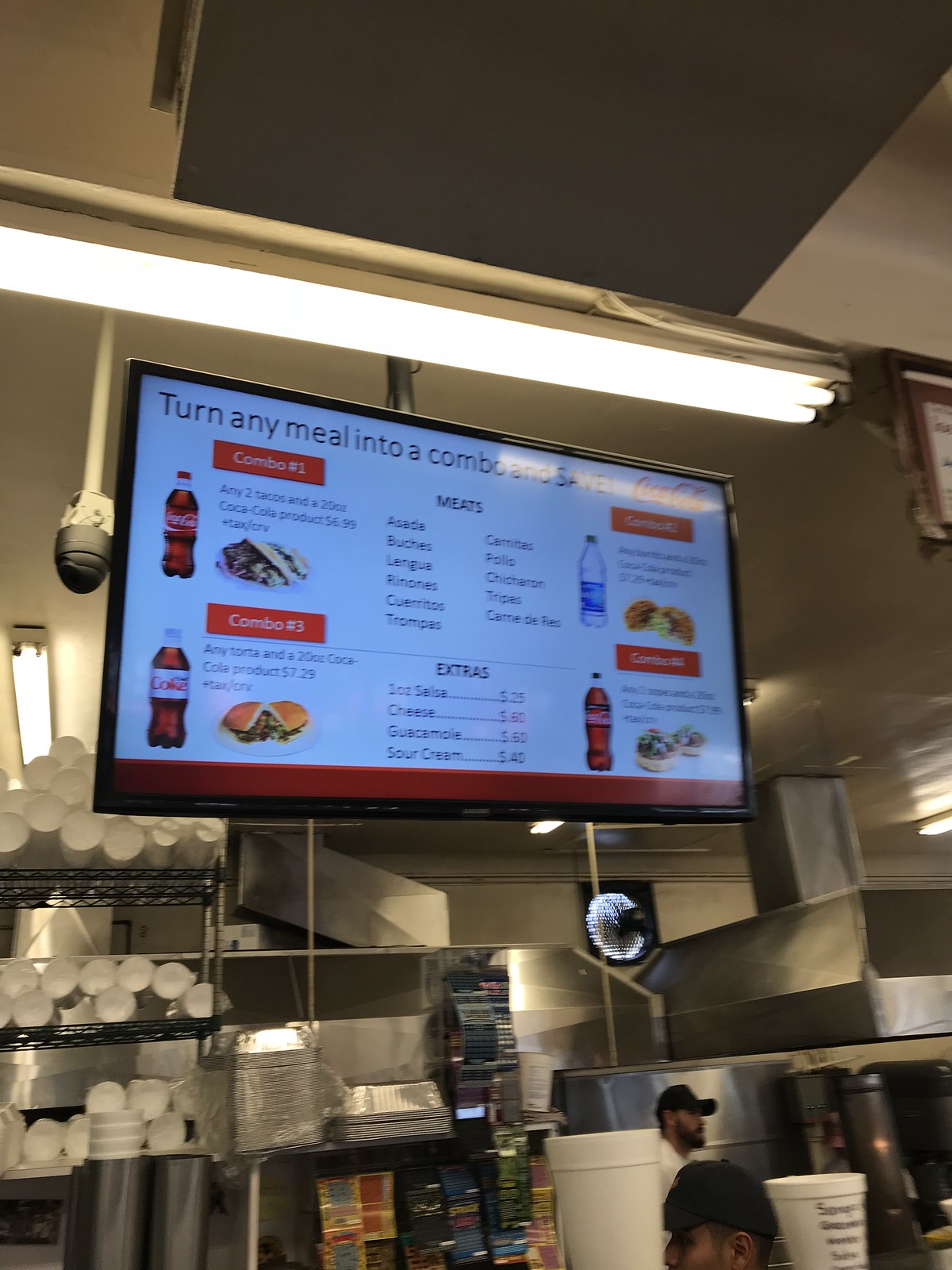The image captures the interior of a fast food restaurant, featuring various elements and details of its design and menu offerings. At the top of the image is a ceiling with a gray box and white sides. Below, there appears to be a curtain that looks rolled up to the right, characterized by its crinkled appearance. Underneath the curtain, there is a long light fixture that is turned on.

Prominently displayed is a large digital menu screen. In black font, the screen advertises, "Turn any meal into a combo meal and save." Towards the right of this message, the traditional red Coca-Cola logo is visible. Below this logo, a red rectangle with white letters reads "Combo Number One," accompanied by black lettering and a picture of a Coca-Cola bottle. Underneath, another red rectangle states "Combo Number Three" in white letters, and again has black lettering beneath it, with what appears to be an image of a cheeseburger and a bottle of Diet Coke.

Further to the right, the menu lists various meats in Spanish, starting with "Pollo." Below the meats section, labeled "extras," there is a long black border and within it, once again, a bottle of Coca-Cola, topped with a bottle of Dasani water.

To the left of the screen, a metal shelf is laden with numerous Styrofoam cups, with Styrofoam lids on the bottom shelf. Behind this, shelving packed with metal trays is visible, adding to the busy and organized atmosphere typical of a fast-food establishment.